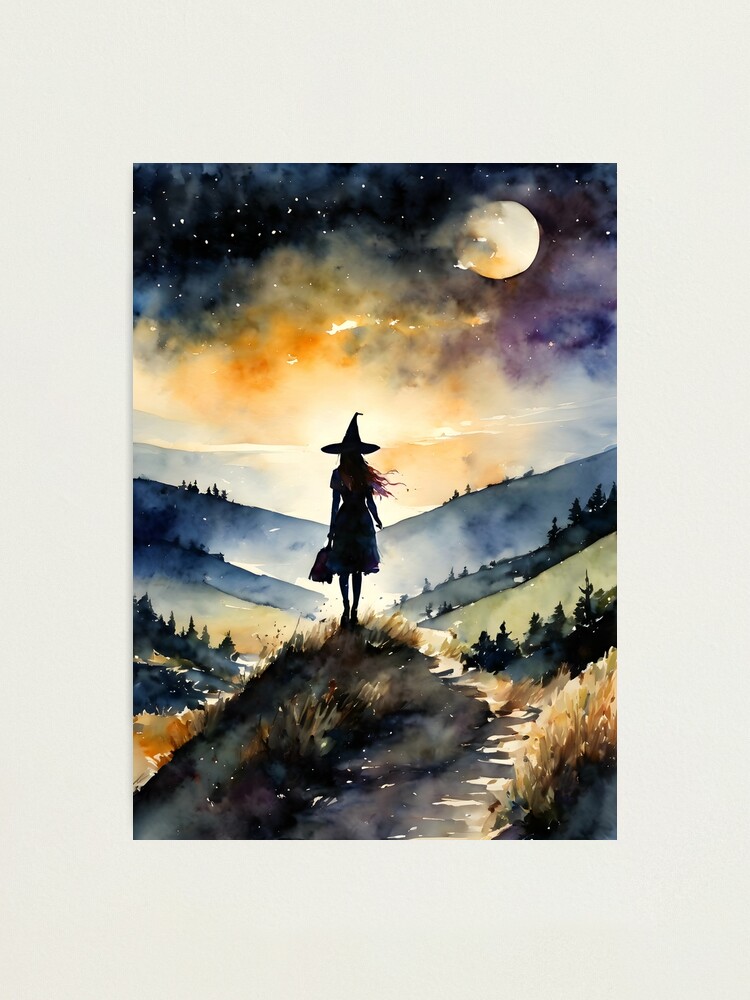This watercolor painting captures a slightly spooky, enchanting night scene. Central to the composition, a silhouetted figure of a girl in a pointy witch hat stands slightly off-center to the left on a grassy, textured hill. She is viewed from behind, with her long hair flowing to the right and a broom carried in her left hand. The sky above is a dramatic blend of dark blue, purple, and orange hues, with stars scattered across a gradient that transitions to a whitish peach sunset. A full moon, partially obscured by wispy clouds of varying colors, illuminates the scene from the top right. Rolling hills of deep blue meld into green, dotted with distant pine trees. Below the central hill, the colors transition smoothly from dark to lighter greens, creating depth. A curved trail leads up to the witch's vantage point, adding movement to this intricately detailed artwork.